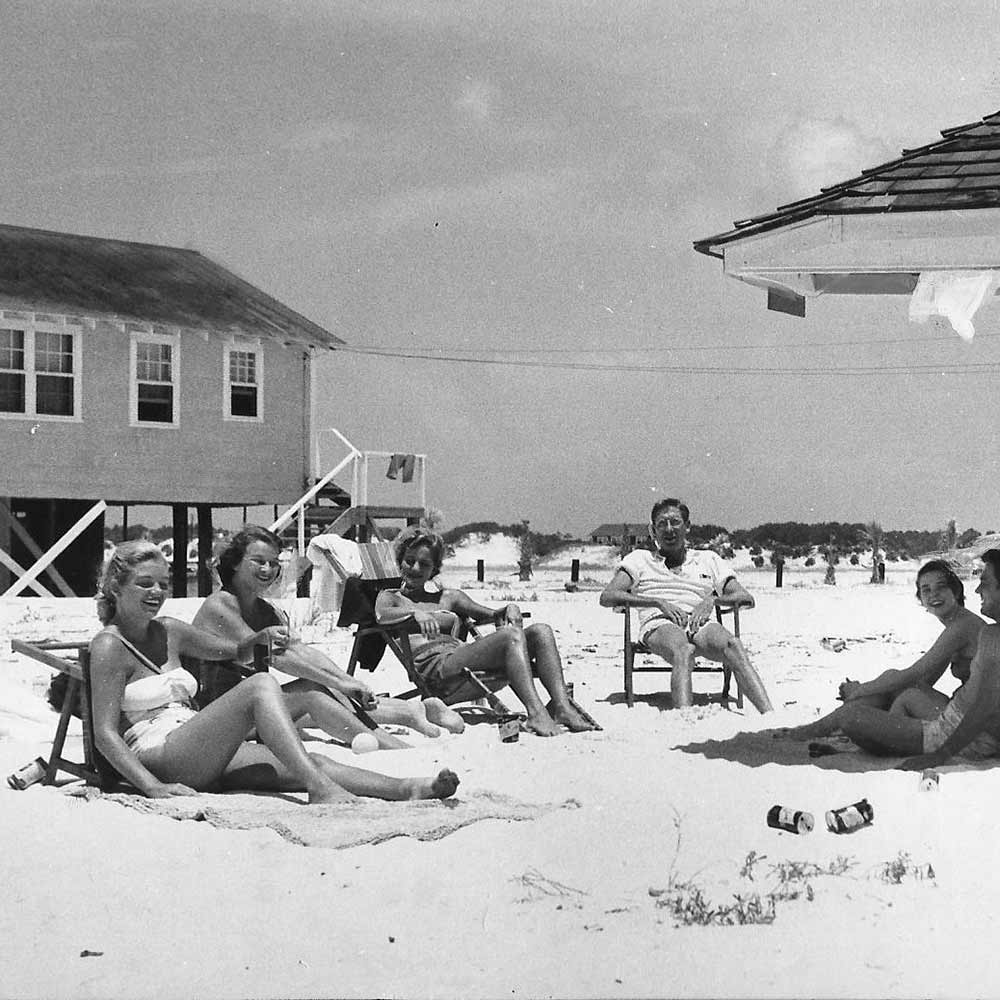This black and white photograph captures a nostalgic beach scene, likely from the past, as evidenced by the vintage style of the buildings and the bathing suits. People are arranged in a semi-circle, lounging on the sandy beach with a few beer cans scattered around, suggesting a relaxed gathering. Central to the image, a tanned blonde woman in a swimsuit sits on a low beach chair beside a gentleman dressed in a white polo and shorts, also seated on a chair. Nearby, another blonde woman with a tie-around-the-neck white swimsuit leans against a beach support with a can beside her, while another individual sits directly on the sand. In the backdrop, a stilted building with a metal roof and paned windows looms, connected by a power line, and reached by a set of stairs. The scene is framed by distant dunes, creating a buffer possibly to the sea, and flanked by a fence and trees, capturing a tranquil moment by the shore under a grey, cloud-dotted sky.